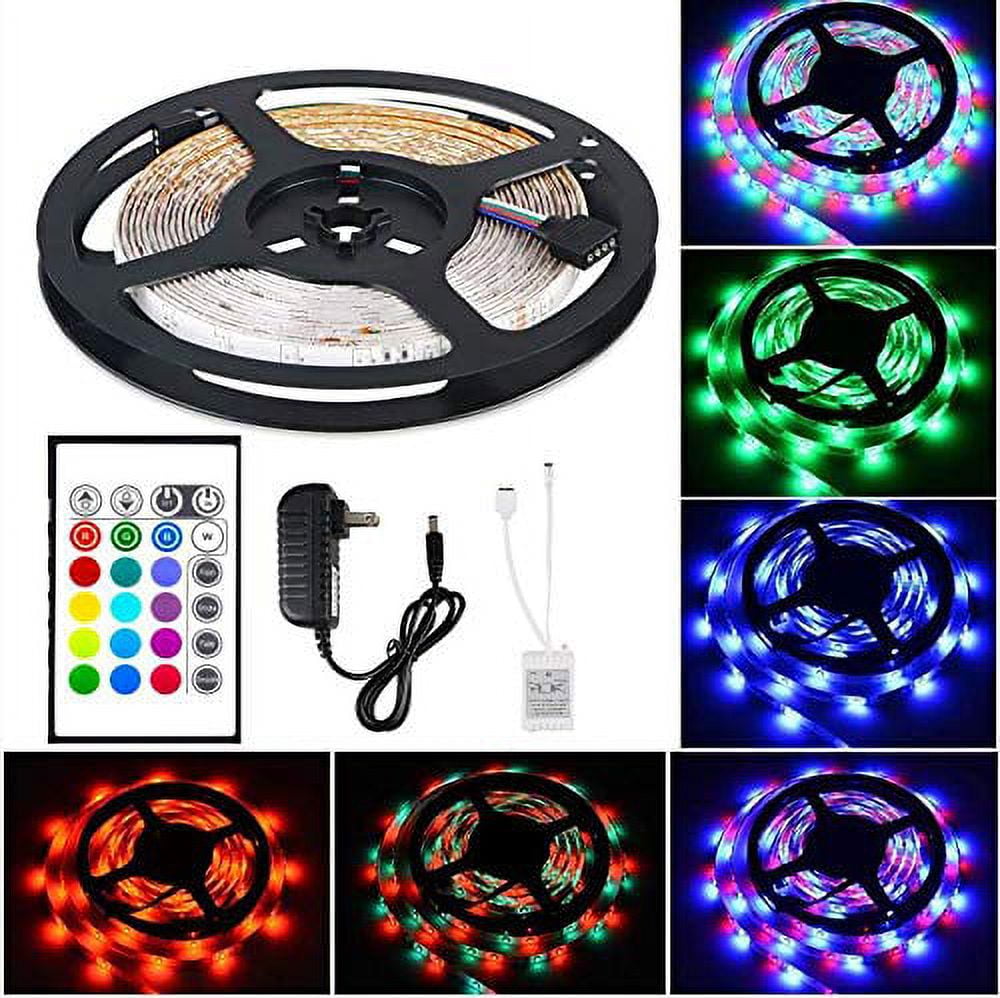The image is a detailed product photo for LED tape lighting, often seen on platforms like Amazon. At the top left, a large central photo displays the main components: a black wheel with the LED tape light coiled around it, an adjacent multi-colored-button controller, a black power plug, and a white adapter. Surrounding this central image in a backwards L-shape are six smaller pictures, each showcasing different color variations of the illuminated tape light. Starting from the bottom left and moving clockwise, the variations include red, red and green, red and white, blue, green, and a mix of red, white, and green. The comprehensive layout of the image clearly demonstrates the product’s versatility and the range of color options available via the remote control.